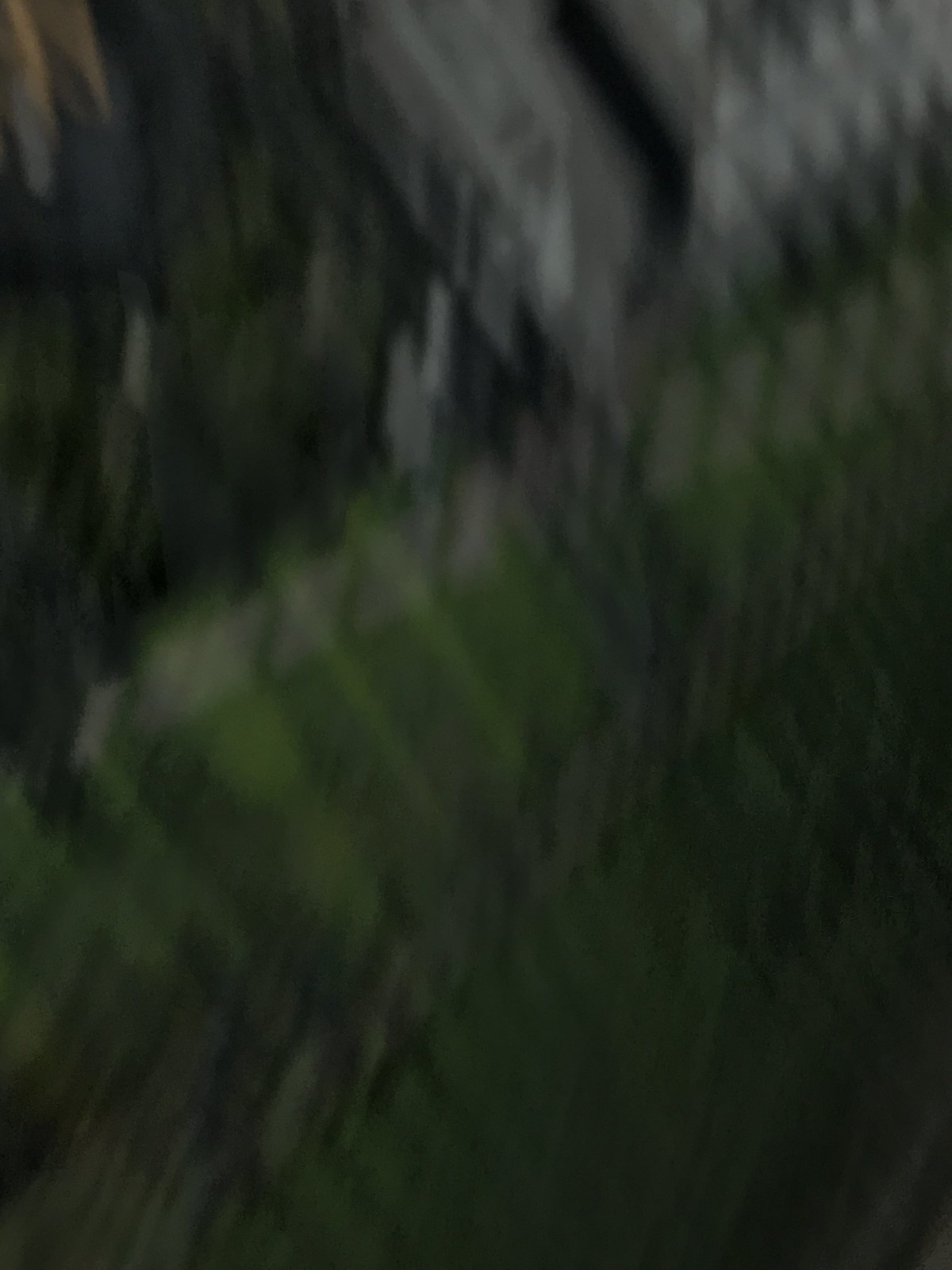This photograph, taken at night, is extremely dark and very blurry, making it difficult to discern precise details. However, several elements can be identified with some effort. The upper left portion of the image appears to show a dark sky or shadowed area, while the upper right part seems to feature a building, possibly white, with indications of a porch or white fence. This area might include trees, bushes, and an entrance with a short staircase. The image is crisscrossed by nearly vertical black lines, suggesting the presence of a dark metal or chain-link fence in the foreground. Below this, at the bottom and center of the image, there's a noticeable patch of bright green grass, and a grayish pathway or sidewalk is visible, running horizontally in the background. There might also be a hint of a gray and white animal or a leg detail in the top middle section, although this could be part of the indistinct and ambiguous features throughout the photograph.